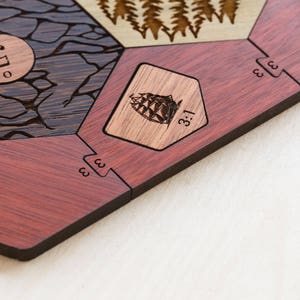The image is a detailed shot of a carved wooden board game reminiscent of Settlers of Catan. The visible portion reveals several intricately interlocking pieces. Notably, there are three reddish-brown pieces, each featuring the number three. One of these pieces shows a square house-like shape carved with an old sailing ship and the inscription "3:1" beneath it.

In the top left corner, a blue piece marked with the number five stands out. Adjacent to it is a beige segment adorned with the carved outlines of trees. The entire board is set against a white background and appears sectioned with a reddish-brown wood grain. The half-visible nature of the board adds a layer of intrigue, with the combination of colored sections, numbers, and carvings suggesting a strategic or decorative purpose.